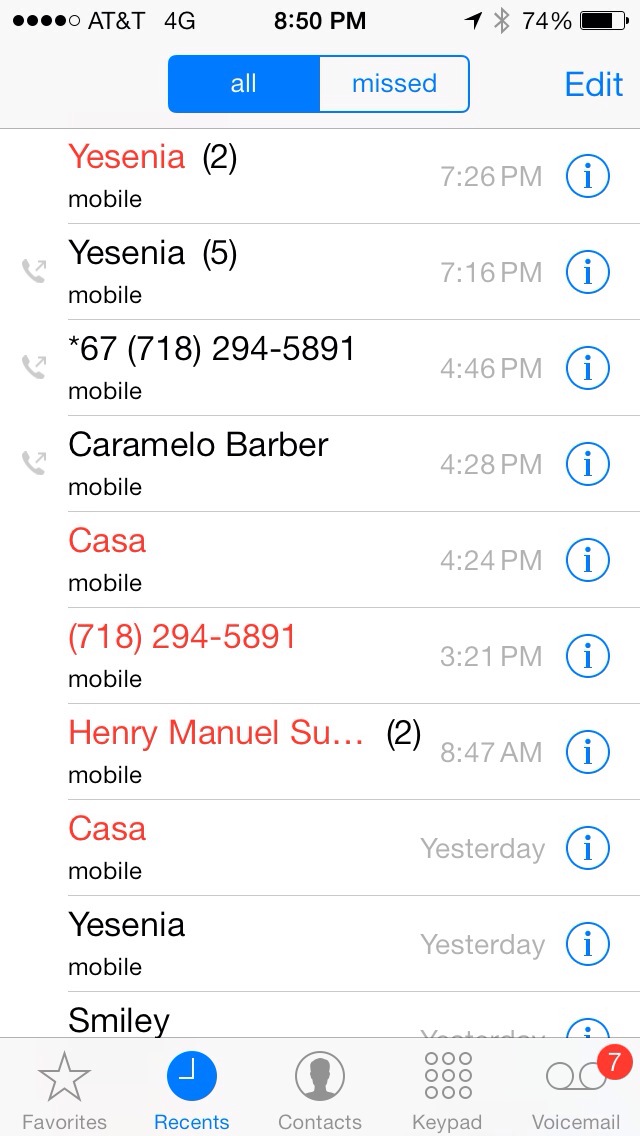This image is a detailed screenshot of the recent call log from an Apple iPhone on the AT&T 4G network, captured at 8:50 p.m. The status bar at the top indicates four out of five signal bars, 74% battery life, and other typical indicators. The user is viewing the "Recents" tab under the "All" category, with "Missed" and "Edit" options available.

The call log reveals a series of interactions throughout the day, including:
- A missed call from Yesenia at 7:26 p.m. and an earlier outgoing call to her at 7:16 p.m.
- Multiple entries from a contact named Yesenia, indicating frequent communication.
- An outgoing call to Carmelo Barbara at 4:28 p.m.
- Missed calls from the number 718-294-5891 at various times, including 4:46 p.m. and 7:24 p.m.
- An outgoing call to Henry Manuel at 3:21 p.m.
- A contact named Casa with entries marked at 8:47 a.m. and yesterday.
- A call from a contact identified as Smiley marked at 7:24 p.m. yesterday.

At the bottom of the screen, the navigation bar shows options for Favorites, Recents (currently selected), Contacts, Keypad, and Voicemail, with an indicator of 7 unheard voicemails. The detailing of times and repeated interactions highlights the call activity and connectivity of the user on this particular day.